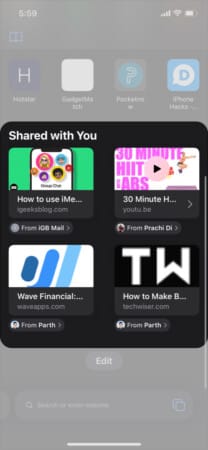This image showcases a slightly blurry screenshot of a smartphone, likely an iPhone, given the visible icon in the background that hints at "iPhone." The main focus is on a modal or pop-up box titled "Shared with You." This box contains four distinct icons or thumbnails, each representing shared content.

The first thumbnail is titled "How to use iMessage," suggesting a guide on using Apple's messaging service. The second icon is labeled "30-minute HIIT apps," indicating a collection or recommendation of high-intensity interval training applications. The third item reads "Wave Financial," likely referring to a financial service or app. The final icon is somewhat ambiguous, displaying "howtomakebee" alongside a logo with "TW." The partial URL "techsomething.com" suggests it might be related to a tech website.

Despite the small and somewhat unclear text, each icon provides a concise glimpse into various topics, ranging from messaging tutorials and fitness apps to financial services and potential tech guides.